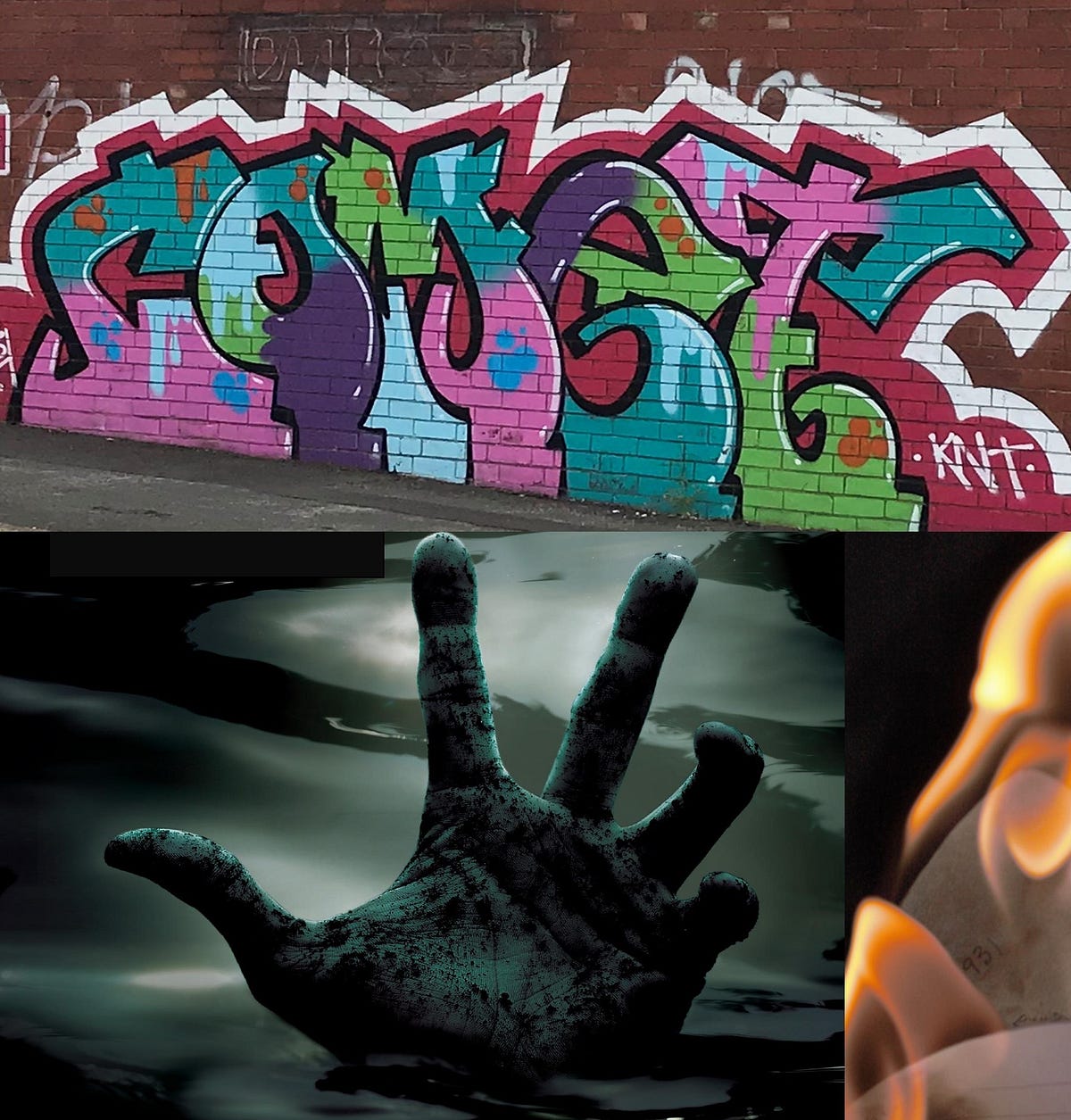In this striking AI-generated artwork divided into three distinct panels, the top section features vivid graffiti on a dark red brick wall. The graffiti prominently displays the artist's initials "KNT" in white amidst an array of bright colors including pink and ocean green, with accents of lime green and purple, all outlined in red with a white border. The middle section portrays an eerie decomposing hand emerging from murky gray water. The hand, dark and ominous, has its four fingers bent and the thumb extended, as if reaching out. The smallest panel on the right contains an abstract composition with shades of orange, tan, and hints of gray, though it remains largely ambiguous in form. This multifaceted piece combines urban street art, unsettling imagery, and abstract design to create a compelling visual narrative.